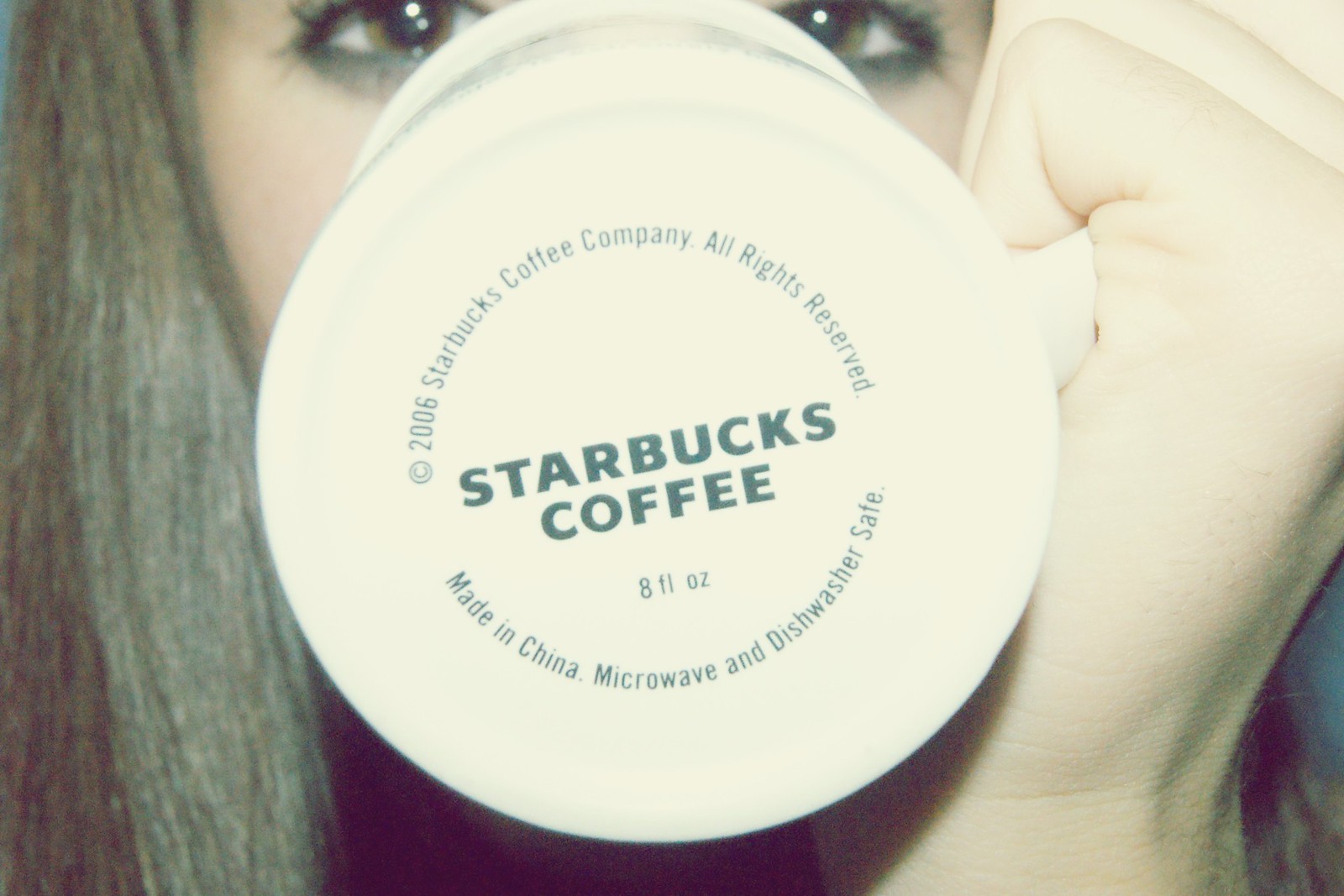The faded photograph, possibly black and white or a highly desaturated color image, features a young Caucasian woman with brown hair and brown eyes, captured as she drinks from a white Starbucks mug. The bottom of the mug faces the camera, displaying the trademark Starbucks Coffee logo in black, surrounded by additional text including "2006 Starbucks Coffee Company, All Rights Reserved, Made in China, Microwave and Dishwasher Safe, 8 fluid ounces." Her left hand holds the mug, obscuring her nose and mouth, while only her eyes and part of her hand are visible. The setting is ambiguous, and the photograph heavily emphasizes the Starbucks branding at the center, making it appear almost like an advertisement.